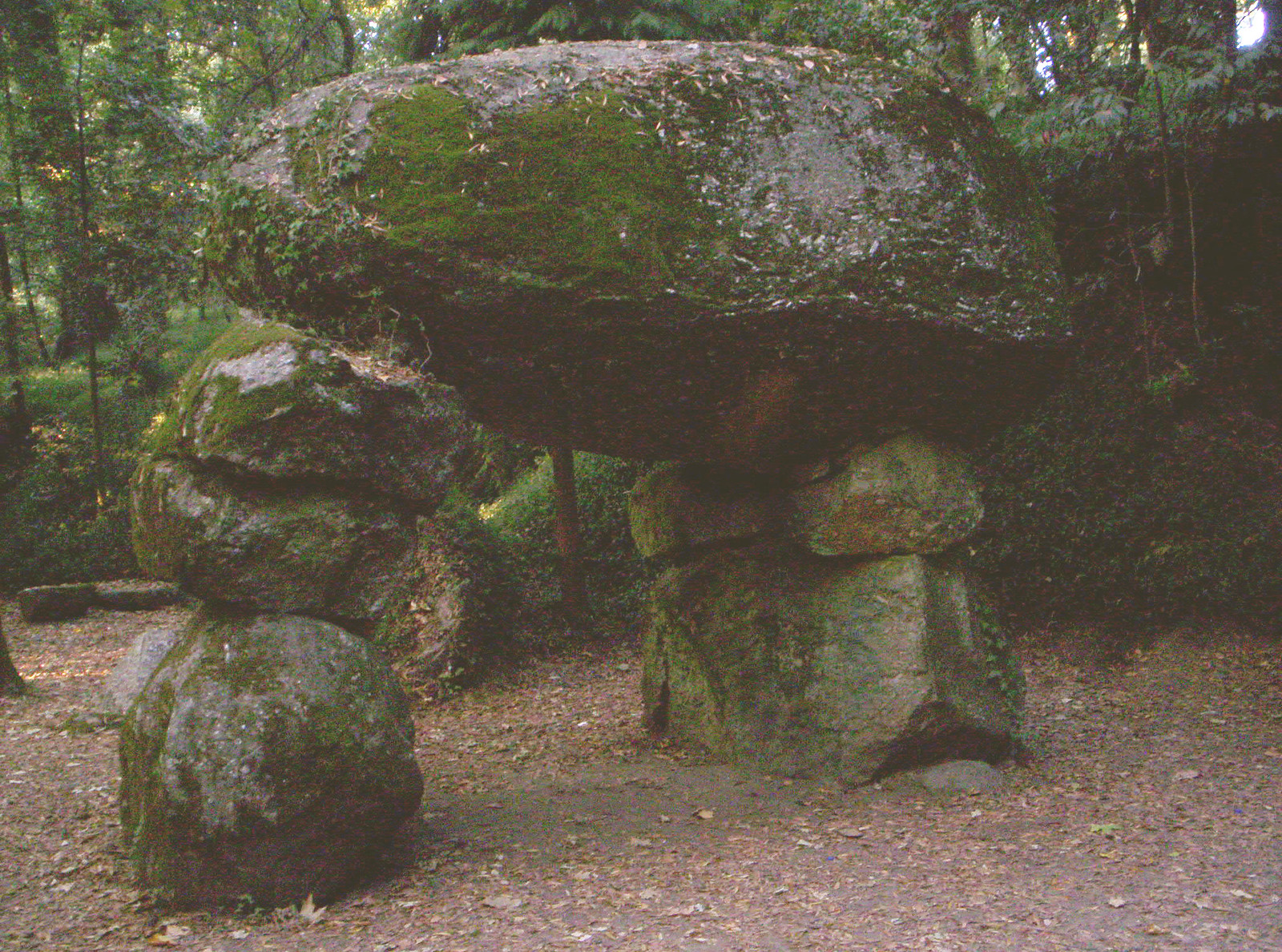The photograph depicts an intricate stone rock formation situated in a forested area. The structure, which appears to be deliberately constructed to resist toppling by predators, consists of seven large rocks covered in thick layers of green moss. It features two distinct columns: the left column comprises three rectangular rocks stacked vertically, while the right column includes a larger spherical base rock with two additional spherical rocks placed on top. Bridging these two columns is a massive horizontal rock, creating a natural archway. The rock formation is set on a brown, leaf-strewn ground, and the background reveals a dense expanse of trees, contributing to a natural, woodland atmosphere. The photograph, although somewhat washed out, highlights the impressive stability and design of the structure amidst the lush greenery and creeping plants of the forest.